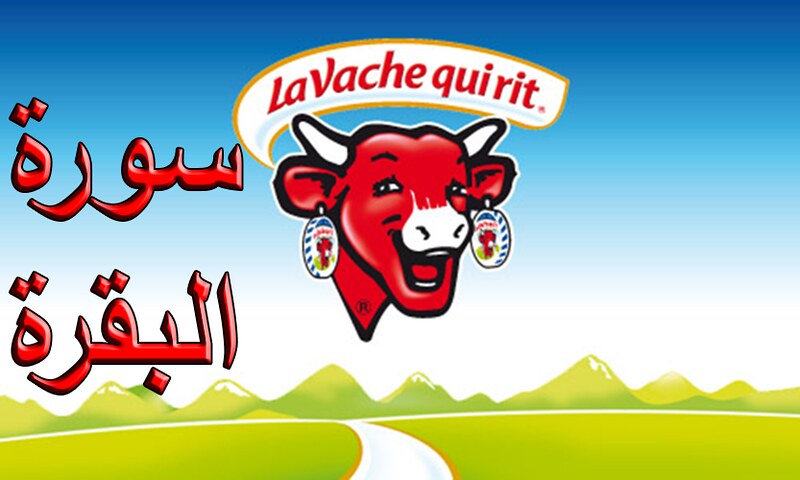The advertisement features a red cow with white horns and a white nose set against a gradient blue sky that transitions to white. The cow's large, expressive face is adorned with earrings that are actually round packages of cheese, each displaying the same image of the cow. Above the cow, in bold red letters on a white background, is the caption "La Vache Qui Rit," with the text appearing in what seems to be Arabic script alongside it. The cow also has an R with a circle around it in black near its neck. Beneath the cow, the landscape includes vibrant green grass, a winding white road, and rolling green mountains, completing the idyllic scene.